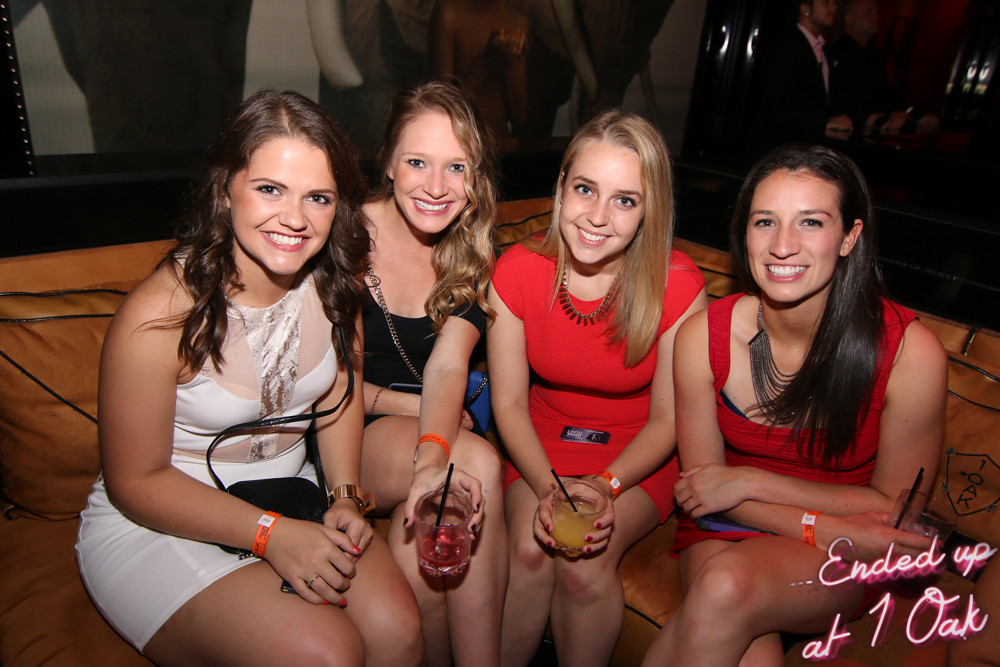The picture features four young women, approximately 25 years old, posing for a group photo while seated on a tan leather couch in a dimly lit nightclub, identified as One Oak by the pink text in the lower right corner. The woman on the far left is wearing a short white dress, accessorized with a black clutch, a red wristband, and has long brown hair flowing over her shoulders. The second woman is in a black top and skirt, holding a drink with a straw in her left hand. She has curly blonde hair and a blue purse. The third woman wears a red dress with a necklace and has long blonde hair. She holds a yellow drink with both hands and has a phone on her lap. The woman on the far right is also in a red dress with a necklace and has long black hair cascading over one shoulder. All four women are smiling, with drinks in hand, giving off a lively and joyful vibe; behind them, other club-goers are faintly visible in the dark background.